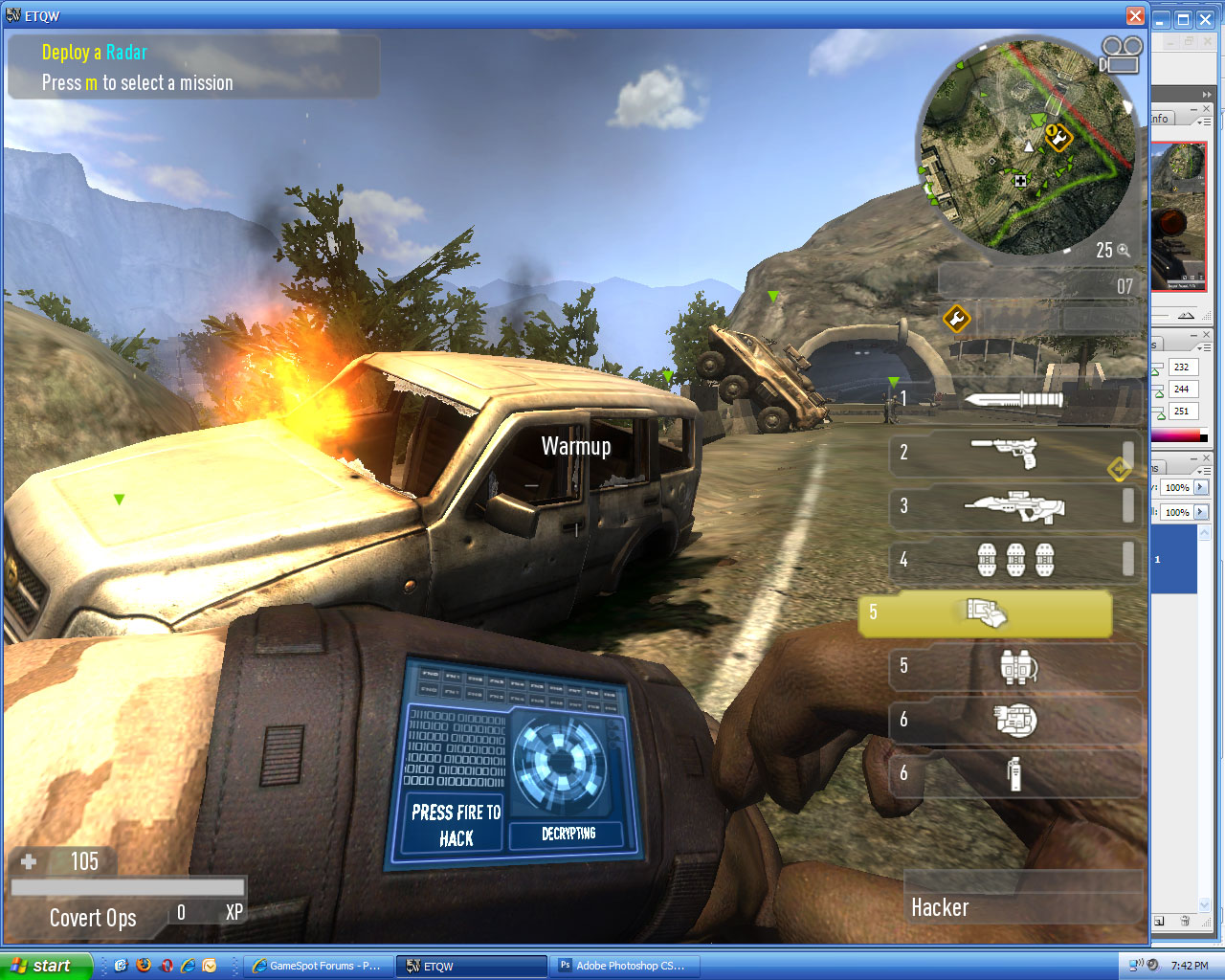The image is a screenshot from a video game on a Windows XP desktop, identifiable by the Start bar at the bottom with Microsoft’s logo and icons for Firefox, Internet Explorer, and Adobe Photoshop CS. The time displayed is 7:42 p.m. In the upper left corner of the gaming window, the letters ETQW appear, with text below instructing to "Deploy a radar, press M to select a mission."

The game itself is set in a 3D world. The player’s perspective shows their left arm, which has a wrist-mounted device displaying the message "Press Fire to Hack" and "Decrypting" alongside binary code (ones and zeros). In the center of the screen, the word “warm up” is visible. To the right, there are selectable icons for various weapons and tools, including a knife, pistol, machine gun, grenades, binoculars, and possibly a fire extinguisher. Nearby, an on-screen map and a video recording button are shown.

The scene within the game is quite detailed. The player appears to be standing on the left fog line of a road that leads through a rocky landscape with a tunnel in the distance. A six-wheeled vehicle is attempting to cross a barrier, and further ahead, a damaged vehicle is on fire, its windows shattered and body heavily battered. The environment includes rugged rock faces and distant mountains under a light blue sky with white clouds.